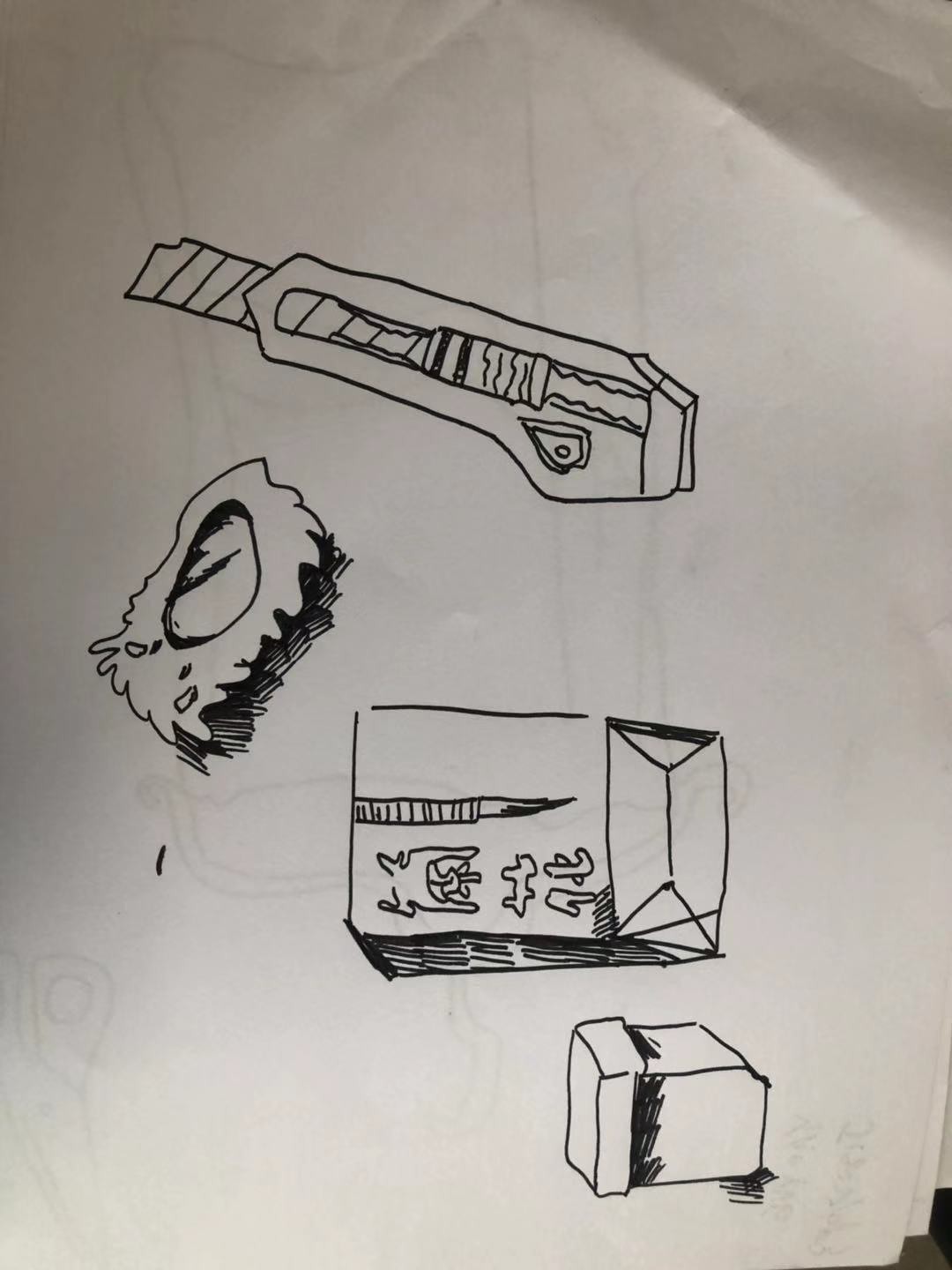This image features a plain white sheet of paper adorned with various doodles made using either an ink pen or a felt-tip marker. At the top of the page, a box cutter is depicted with its blade extended to the left. Directly below the box cutter is an upside-down sketch of what appears to be a fuzzy animal with its mouth wide open. Further down and to the right, there is a drawing of a folded paper bag with a pen drawn emerging from the top, pointing downward. Below this, a file box with a lid is illustrated, positioned on its side and directed towards the left. Additional sketches can be faintly seen through the paper from the reverse side, suggesting more doodles on the back.